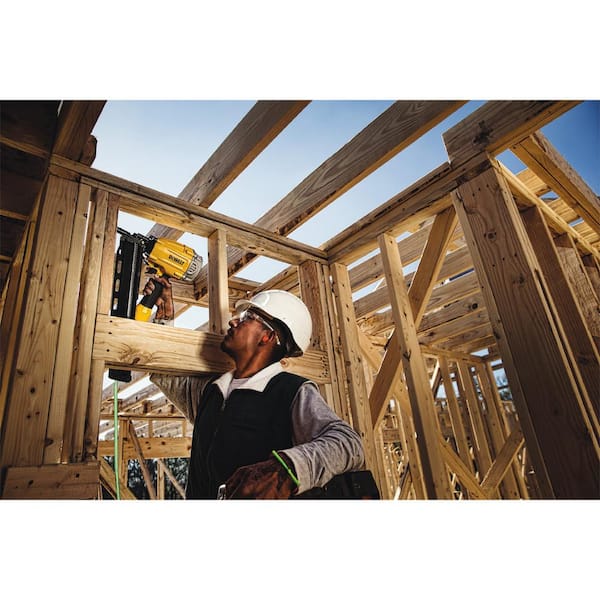The image captures a close-up, daytime view of a construction site where a house is being framed. The photographer's angle is slightly upwards, revealing the blue sky above the wooden framework of walls, doorways, and rooftops. Trees are visible in the bottom left and center-right of the frame. The primary focus is a dark-skinned man, standing under the wooden beams of the structure. He's dressed in standard protective gear: a white hard hat, safety goggles, red ear protection, and a gray long-sleeve shirt under a black vest with a white collar. He is using a large DeWalt hand tool, either a drill, air gun, or nail gun, to work on a window frame. His arm extends outward under a beam, suggesting he might be manipulating the frame or carrying a tool bag. The overall scene highlights the active and intricate process of home construction against a clear, sunny sky.